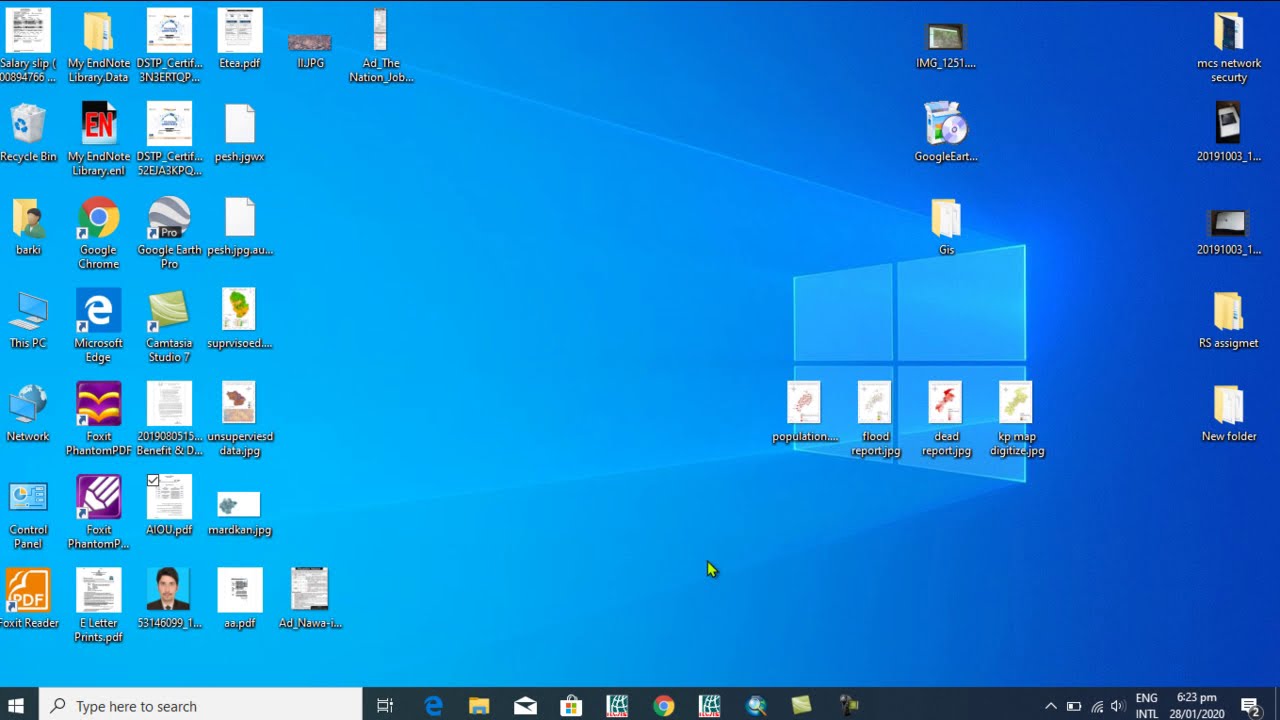This image is a screenshot of a computer's home screen. The background features a gradient blue transition from light blue on the left to darker blue on the right, with a subtle illuminated Windows logo in the backdrop. The bottom edge of the screen is lined with a black toolbar, containing icons for Internet Explorer, Google Chrome, and various other applications. On the far left of this toolbar lies the main Windows navigation button and a white rectangular search bar with a magnifying glass icon and the text "Type here to search." Moving rightward, additional small icons represent various system interactions.

On the bottom right corner, the date and time are displayed along with icons indicating the health and status of the PC, such as Wi-Fi, battery life, and Bluetooth connection. The left-hand side of the screen is populated with numerous icons, including those for Microsoft Edge, Google Chrome, and Google Earth Pro, arranged in rows—some rows holding as many as six icons, while others hold four or five. In the center, a smaller cluster of icons is vertically aligned, consisting of about three rows, each with approximately four icons horizontally. The right-hand side of the screen similarly holds several folders and icons, including one labeled "New Folder," organized in a descending vertical row of five icons.